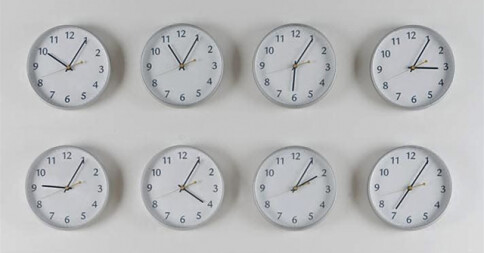This image features eight identical white clock faces with black numerals, each telling a different time. The clocks are mounted on a clean, white rectangular background, creating a minimalist and cohesive aesthetic. The times displayed on the clocks range systematically. The first clock on the left shows 10:00, while the last clock on the right reads 7:05. The varying times suggest a possible puzzle or sequence that invites viewers to decipher their meaning.